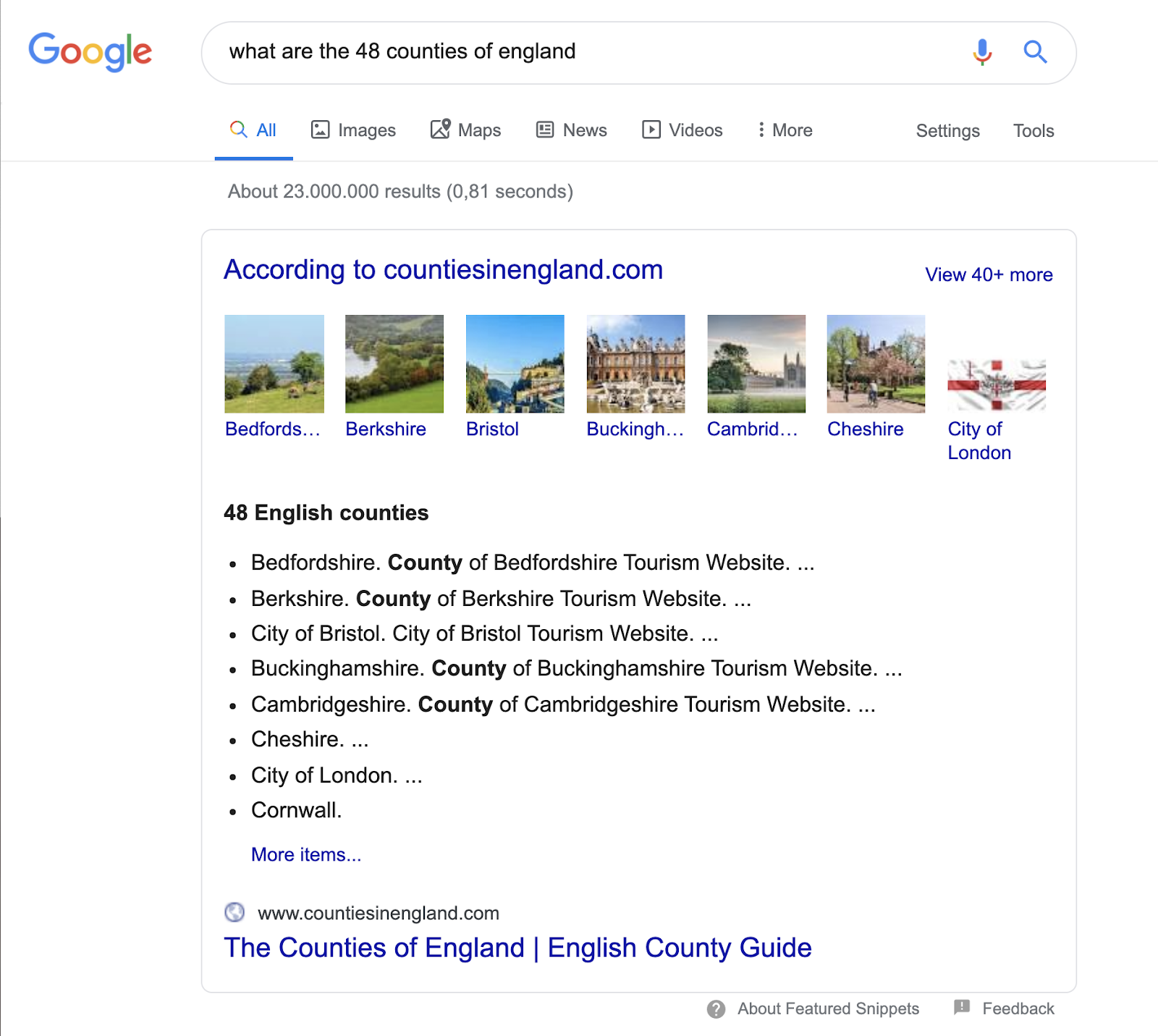The image displays a Google search results screen against a white background. In the upper left corner, the iconic Google logo appears in its usual vibrant colors: blue, red, yellow, blue, green, and red. The Search bar contains the query "what are the 48 counties of England." 

Just below the search bar, there are several options for refining the search, with the first option "All" highlighted in blue and underlined. Next to it, from left to right, are other options labeled as "Images," "Maps," "News," "Videos," "More," "Settings," and "Tools."

Further down, a blue text citation reads, "According to countiesinengland.com." Directly below this, there are miniature images or thumbnails depicting various English counties. Following this, in black text, it states "48 English counties," accompanied by a concise bullet list naming counties. The top entries in this list include Bedfordshire, Berkshire, and City of Bristol.